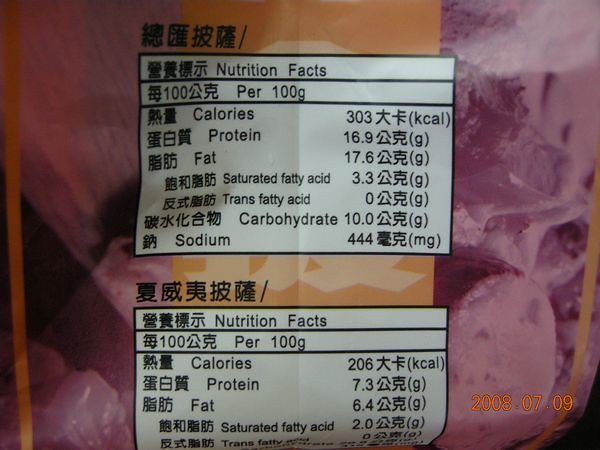The image features a label with various text elements written predominantly in Asian characters. Prominently displayed at the top is a large white box outlined in black containing the words "Nutrition Facts" in bold black letters. Just below this headline, the text specifies "per 100 grams," followed by nutritional details provided in both Asian characters and Arabic numerals. Key nutritional information outlined includes:

- Calories: 303
- Protein: 16.9g
- Fat: 17.6g
- Saturated Fatty Acids: 3.2g
- Trans Fatty Acids: 0g
- Carbohydrates: 10.0g
- Sodium: 444mg

Below this main label, there is another section with more nutritional data where different values are presented:

- Calories: 206
- Protein: 7.3g
- Fat: 6.4g
- Saturated Fatty Acids: 2.0g

The remaining values on this secondary label are cut off and not fully visible.

The background of the image features a blend of purple and orange shades, possibly hinting at a product like a fruit drink or another consumable item. Near the bottom of the label, an orange section with tiny printed numbers displays "2008 07 09," likely indicating a date.